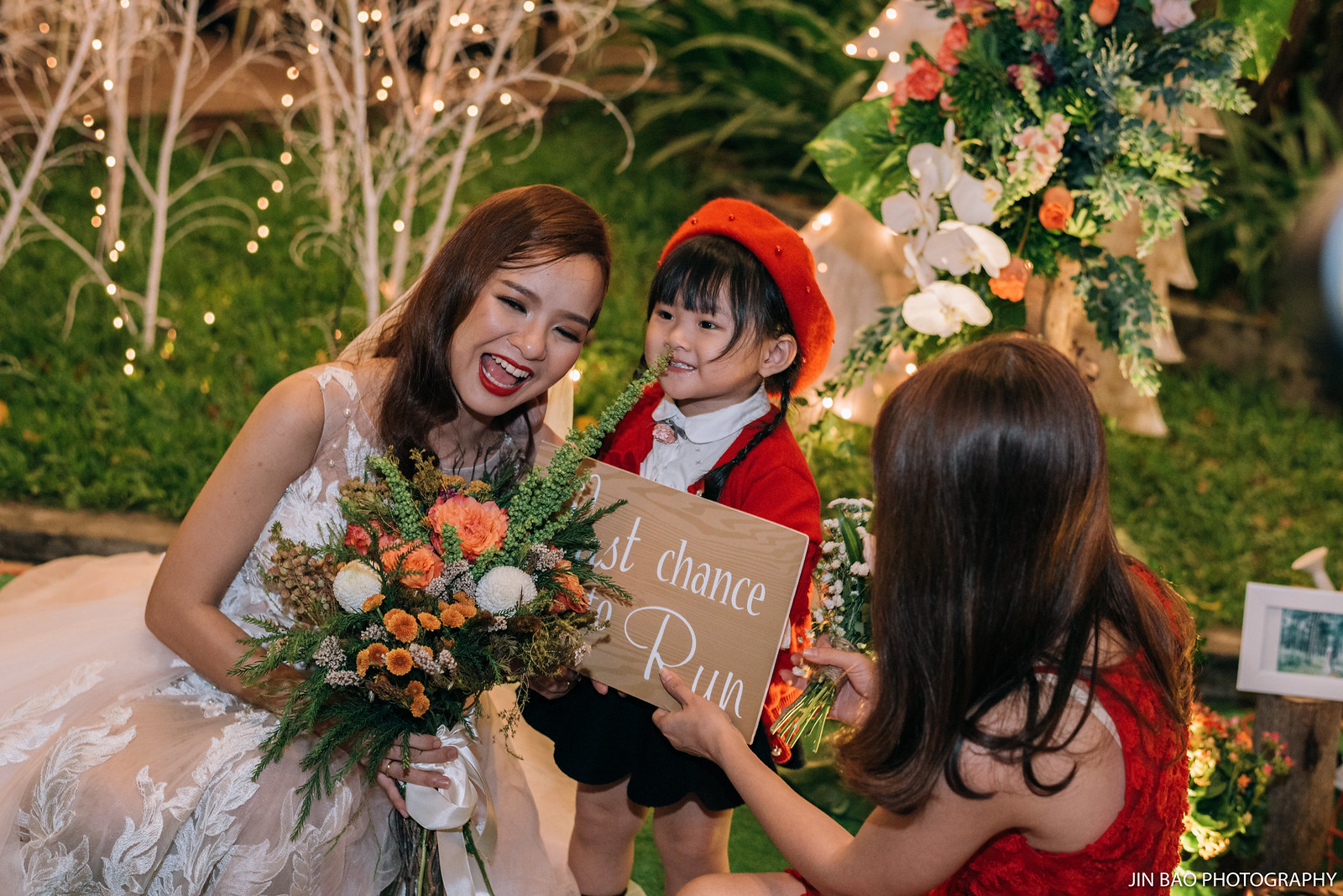The image captures an outdoor evening wedding scene, centered around a joyful bride in a white dress with brown hair and red lipstick, holding a vibrant bouquet of orange, pink, and green flowers. Beside her stands a little Asian girl with black braided pigtails, wearing a red beret, black skirt, white blouse, and red sweater. The girl is helping to hold a wooden sign emblazoned with "Last Chance to Run" in white letters. To the right, another woman with long brown hair, clad in a red dress, assists with the sign. The backdrop is an ornate display of lit-up trees, flowers, bushes, and various decorative items, with the lush green grassy ground below hinting at a serene, twilight atmosphere. The setting is accentuated with hanging lights that illuminate the scene, enriching the visual charm of the wedding ambiance.